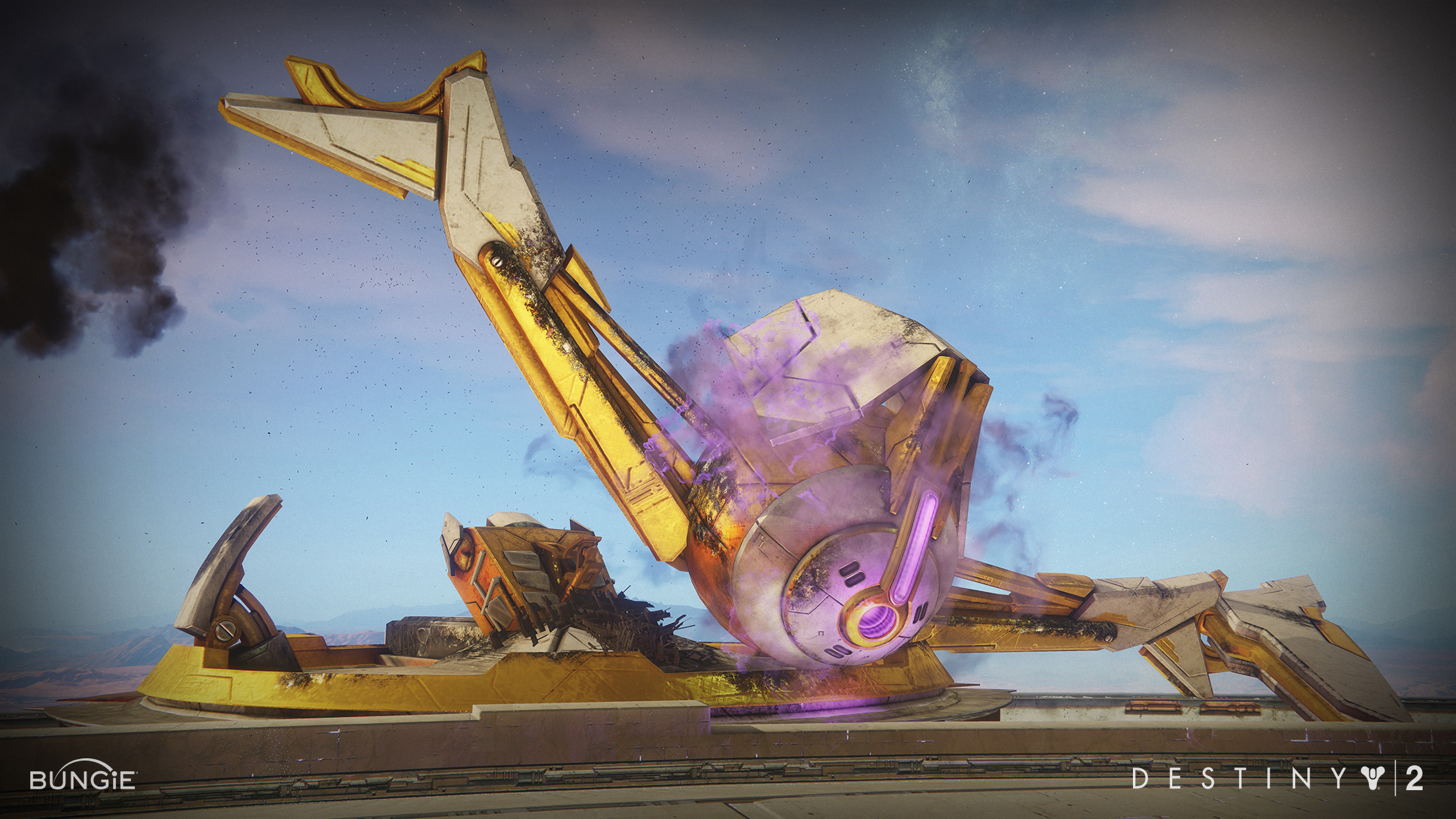The image depicts a large, yellow, sci-fi vehicle that resembles a hybrid between a bulldozer and a spacecraft, appearing to be a downed or crashed ship emitting both black and purple smoke. The vessel has two yellow arms with white tips and is surrounded by a bright blue sky with some white clouds. Illuminated by purple lights, parts of the machinery look damaged, with rust spots visible on its wings. On the lower left, the image is signed with "Bungie," and on the lower right, it features the "Destiny 2" logo, indicating it is likely related to the video game "Destiny 2." The overall scene portrays a futuristic, large piece of equipment in ruins.